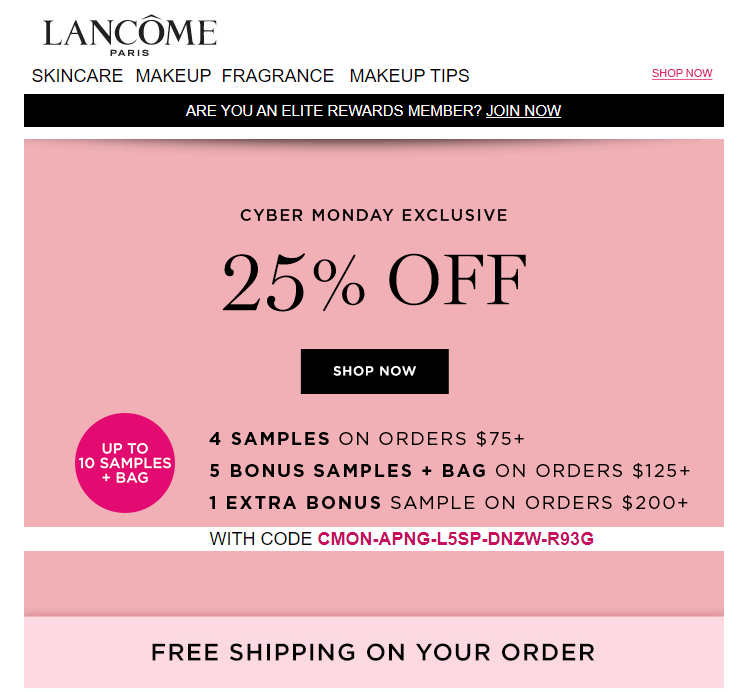The image displays the homepage of the Lancôme Paris Makeup Company website. 

Starting at the upper left corner, the word "Lancôme" is prominently featured in black font, with "Paris" written in smaller font beneath it. Moving from left to right, the main navigation menu includes categories like "Skincare," "Makeup," "Fragrance," and "Makeup Tips," all in black text. On the far right, there is a striking pink link that says "Shop Now."

Below the navigation menu, a black bar stretches horizontally across the page, featuring white, uppercase text that reads, "ARE YOU AN ELITE REWARDS MEMBER? JOIN NOW."

The main section of the page has a light pink background. Centrally positioned, though not in the exact middle of the image, is the text "Cyber Monday Exclusive" in smaller black font. Below this, "25% off" is displayed in large, bold black letters. Beneath this offer, there is a button labeled "Shop Now" in black.

Further down, three lines of promotional text are listed:
1. "Four samples on orders $75+."
2. "Five bonus samples plus bag on orders $125+."
3. "One extra bonus sample on orders $200+."

To the left of these promotional offers is a darker pink circle with the text "Up to 10 samples plus bag" written in white.

At the very bottom of the section, a white bar spans the width of the page with the text "WITH CODE" in black capital letters, followed by a long, random string of digits in pink. The bottom line of the image announces "Free shipping on your order."

In summary, the image is a promotional webpage from Lancôme Paris highlighting an exclusive Cyber Monday deal with various incentives for different order amounts.